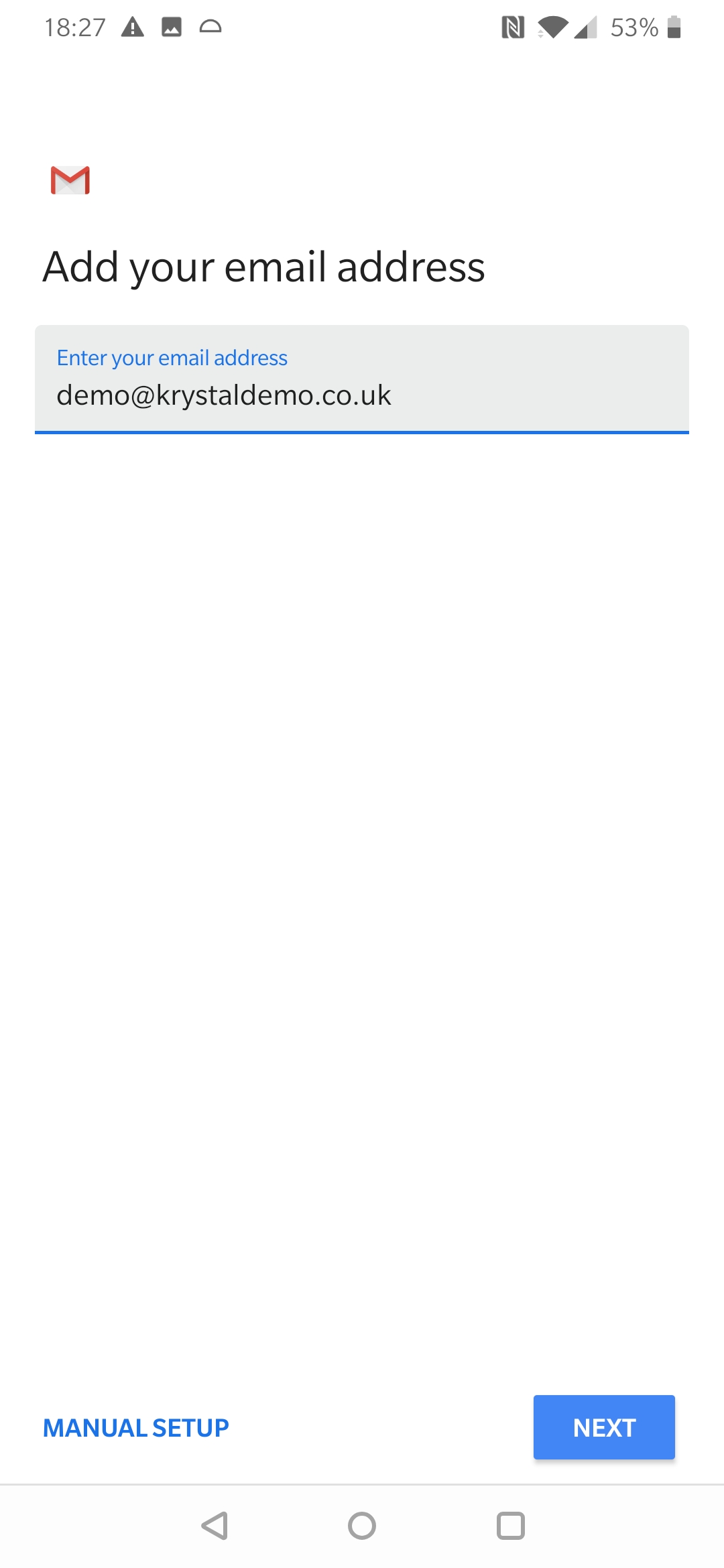This image is a detailed screenshot of a cell phone user interface, featuring a predominantly white background with a light gray strip. The time, displayed in black at the upper left corner, reads "18:27." The top right corner shows reception bars and a battery icon that indicates 53% charge. Various application icons are scattered across the top.

Beneath these indicators is the Gmail app interface. Iconography includes the recognizable Gmail logo—an envelope with a red "M." Below, black text prompts users to "Add your email address."

A light gray rectangle beneath this text contains a blue text prompt: "Enter your email address." Below this, black text displays the email address "demo@krystaldemo.co.uk," followed by a horizontal blue line.

The interface continues with a white background dominating the middle portion. At the bottom, on the left-hand side, blue text in all capital letters reads "MANUAL SETUP," while on the right-hand side, a blue rectangular button with white capital letters reads "NEXT."

Further down at the very bottom of the screen, three navigation icons are visible: a left-facing triangle, a circle in the center, and a square on the right.